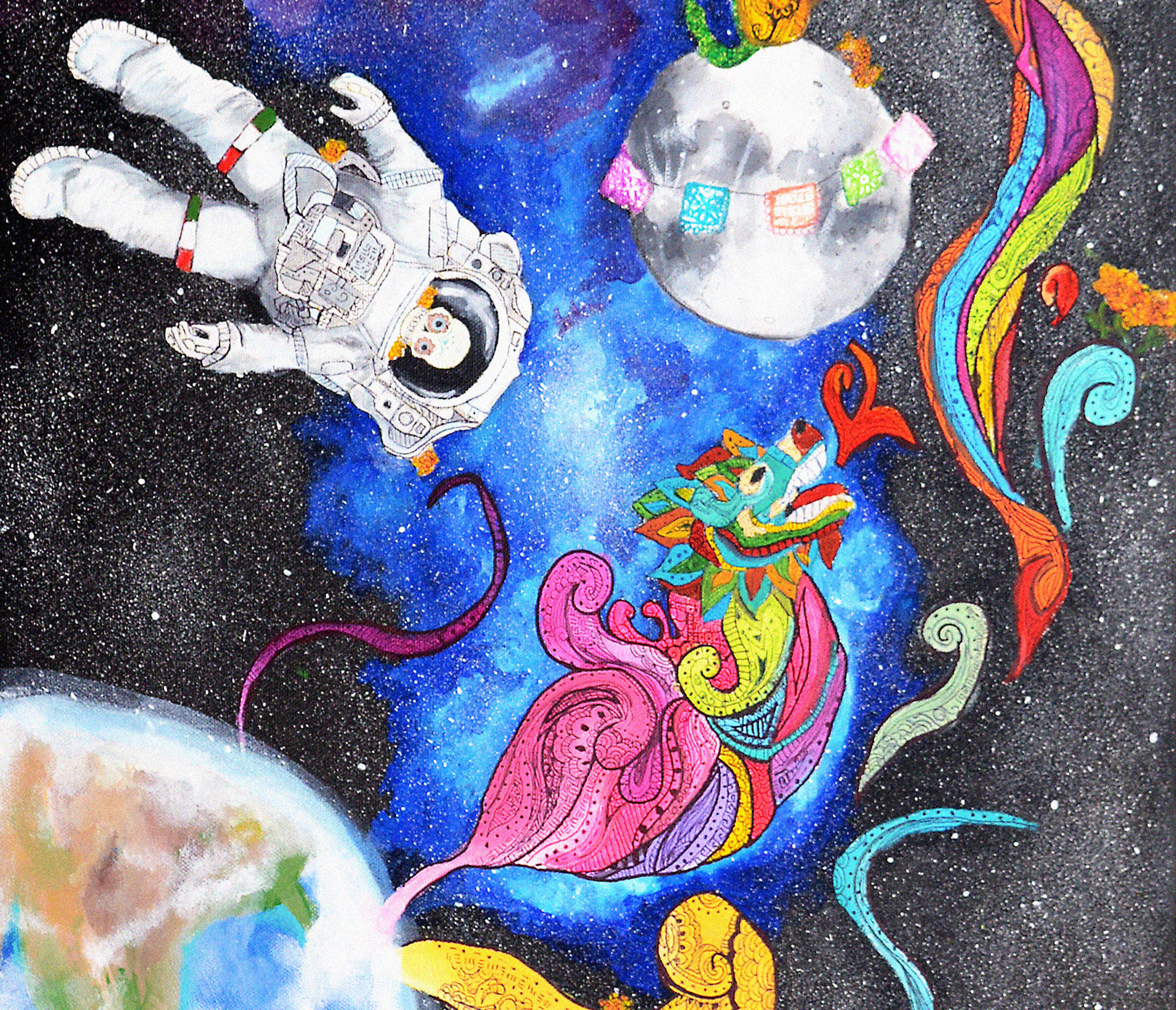This surreal painting, likely done with watercolors in various spots, presents a vibrant and fantastical depiction of outer space. The upper left corner features an astronaut with a skull for a face, eerily complete with eyes. The astronaut's knees are adorned with green, white, and red bands, reminiscent of flags, and it's surrounded by an ambiguous orange hue near the neck and left shoulder. Dominating the scene just below and to the right of center, a large Chinese dragon breathes fire despite the space setting. This dragon is decorated in pastel colors with a paisley design. The Milky Way, depicted in a blue splotchy pattern, stretches from top to bottom in the background, against which both the astronaut and dragon stand out.

The Earth is visible in the lower left, largely obscured by clouds but revealing a glimpse of North America. Emerging from the Earth is a large purple tentacle-like form that touches the Milky Way. Additionally, the painting is detailed with various swirling patterns in multiple colors: a yellow swirl under the dragon, a blue one in the lower right, a short green one above that, a long multicolored one to the left, and a small red one, along with a blue one with two flowers coming out of it on the right side.

There is a moon situated slightly to the right of center, encircled by a sequence of colorful flags in pink, blue, orange, green, and a lighter pink. Atop the moon, there are two indistinct orange forms, possibly cats, and a green object with a blue center. This modern, professional-looking painting, bursting with color and imaginative elements, could make an excellent mural due to its vivid characters and intricate shades.